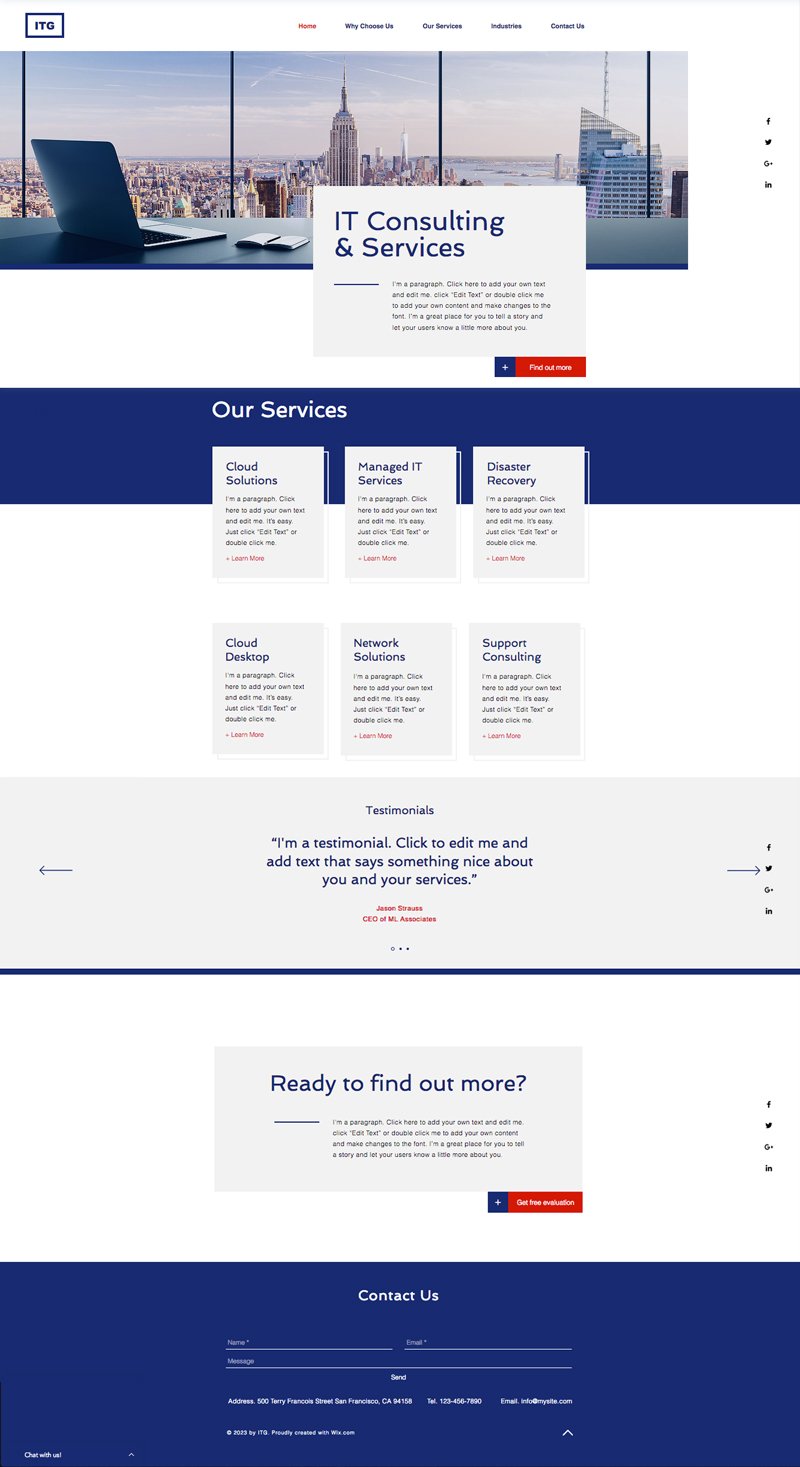The image displays the detailed layout of a business webpage for ITG. Positioned in the top-left corner, ITG's logo appears in a blue font within a box outlined in blue. Adjacent to the logo, navigation tabs such as Home, Why Choose Us, Our Services, Industries, and Contact Us are aligned horizontally. The Home tab is distinctly highlighted in red, while the remaining tabs retain a standard color.

Dominating the background, a panoramic view of the New York City skyline as seen from an office penthouse sets a sophisticated tone. Overlaying this image, a semi-transparent gray box reads "IT Consulting and Services," with a prominent red "Find Out More" tag located at its bottom right corner.

Below the skyline image, a blue stripe housing the white text "Our Services" introduces a grid of six gray boxes detailing the offered services:
- First row: Cloud Solutions, Managed IT Services, Disaster Recovery.
- Second row: Cloud Desktop, Network Solutions, Support Consulting.

Further down, a testimonial from Jason Strauss, CEO of ML Associates, adds credibility to the page. Following this, a gray box titled "Ready to Find Out More" includes a red "Get Free Evaluation" tag, inviting user engagement.

The footer, shaded in navy blue, features a 'Contact Us' section complete with fields for Name, Email, and Message, as well as a centrally positioned 'Send' button. Additionally, it provides the company’s address (500 Terry Francois Street, San Francisco), telephone number, email, and a copyright statement.